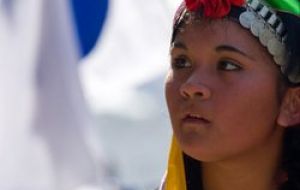This close-up photograph captures a young girl prominently positioned on the right side of the frame. She has olive or light brown skin and a neutral expression, with her mouth slightly open as she gazes to her left. The headdress she wears is intricately designed, featuring circular silver discs draped from a silver band, a striking red flower in the center, and a green ribbon emerging from the upper right corner near her temple. A touch of yellow cloth is visible below her chin on the left. The blurred background to the left of the image includes indistinct white shapes, a blue area at the top, and smudges of black near the bottom, making it difficult to discern specific details. The photograph's quality is not high definition, which adds to the blurriness of the background and the soft focus on the girl and her elaborate headdress.